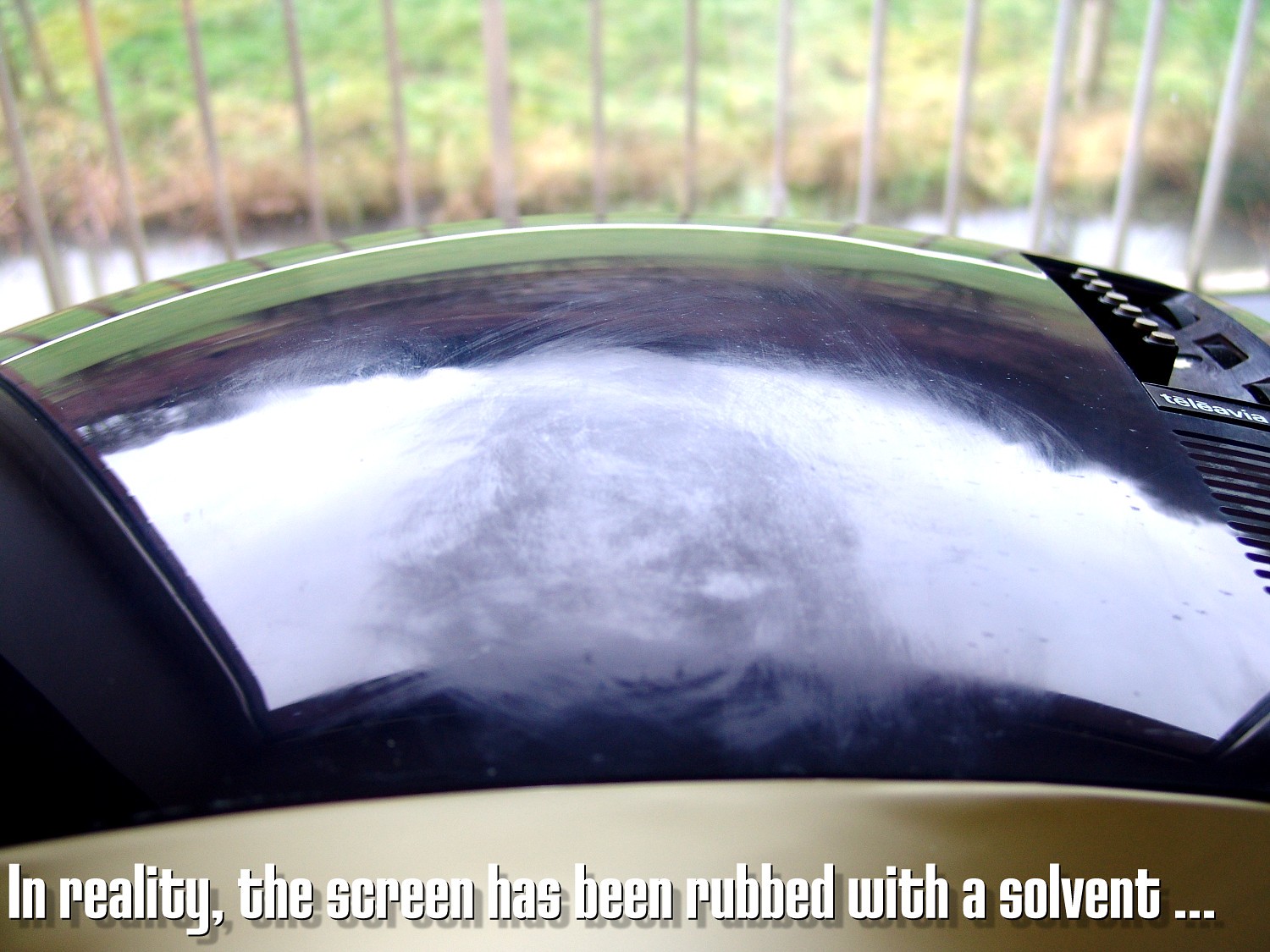The photograph captures an extreme close-up of an old CRT television laying on its side on a porch. The screen is dominated by an extensive network of scratches and smudges, highlighted by the light cascading across its surface. The television’s speaker is visible to the right of the screen, accompanied by several knobs. The background includes hints of a fence and a lawn, with white lines that could be part of a shade or fencing. The television’s top reflects light with a shiny chrome-like surface, and there are buttons visible, suggesting a user interface. At the bottom of the image, a caption in bold white print reads: "In reality, the screen has been rubbed with a solvent..." suggesting that the smudges and scratches are the result of an attempted cleaning.